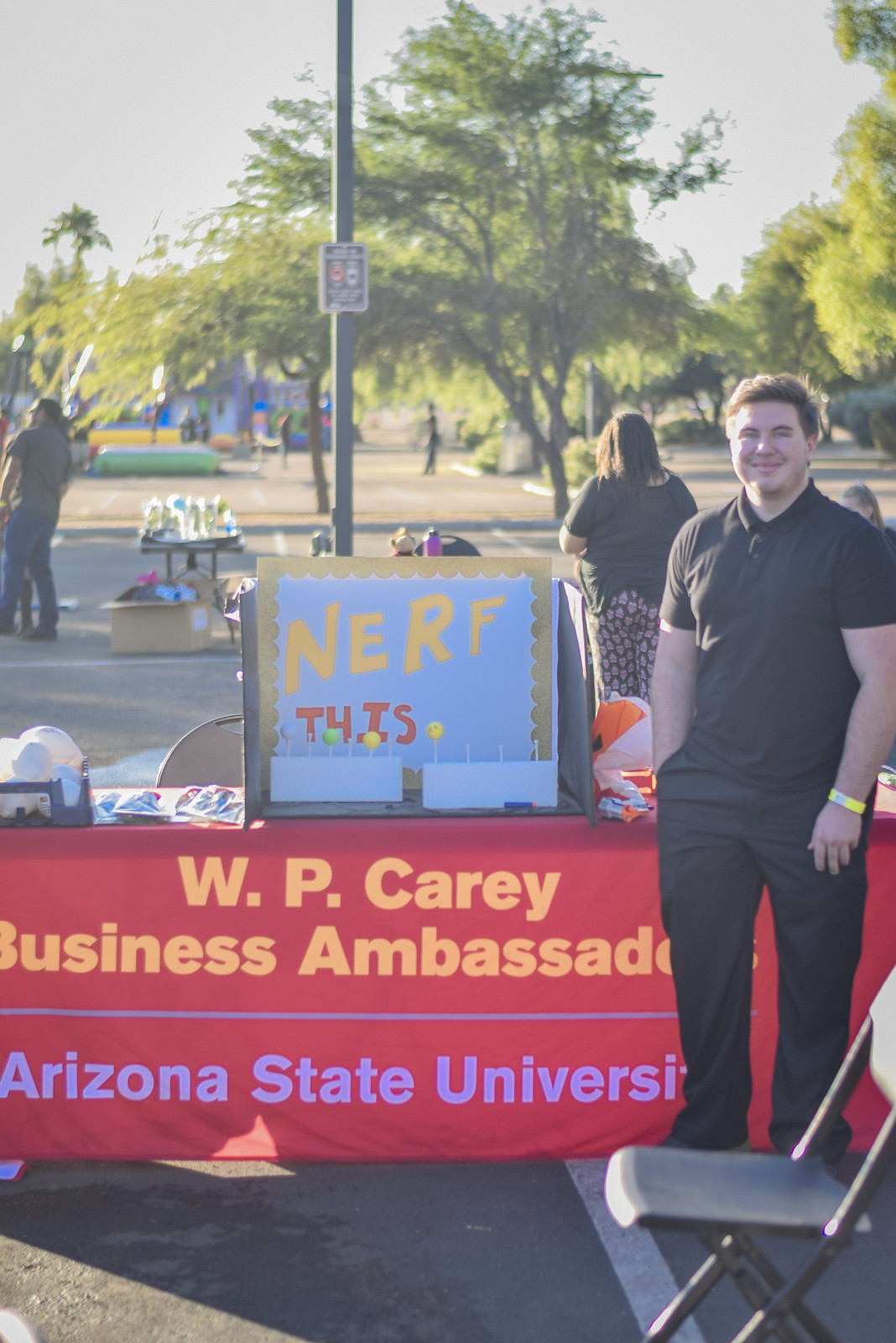The image is a vibrant color photograph taken outside on a sunny day in a parking lot, though the sky appears grayish-blue. There is a young Caucasian man with short dark hair, dressed entirely in black — a black t-shirt and black dressy pants. He stands directly in front of a long table draped with a red cloth, which is inscribed with “W.P. Carey Business Ambassador, Arizona State University.” The man, who is smiling at the camera, has his right hand in his pocket and a blue and yellow bracelet or watch band on his left wrist.

In front of him, there's a black folding chair and on top of the table are various objects, including an orange and white ball and a blue and white ball. Additionally, a sign reads “NERF THIS!” There are more people and stands further in the distance, all set up in the parking lot marked with white-lined spaces and illuminated by streetlights. Surrounding the parking lot are green trees, adding a touch of nature to the urban setting. The overall atmosphere suggests a lively outdoor event occurring in the middle of the day.